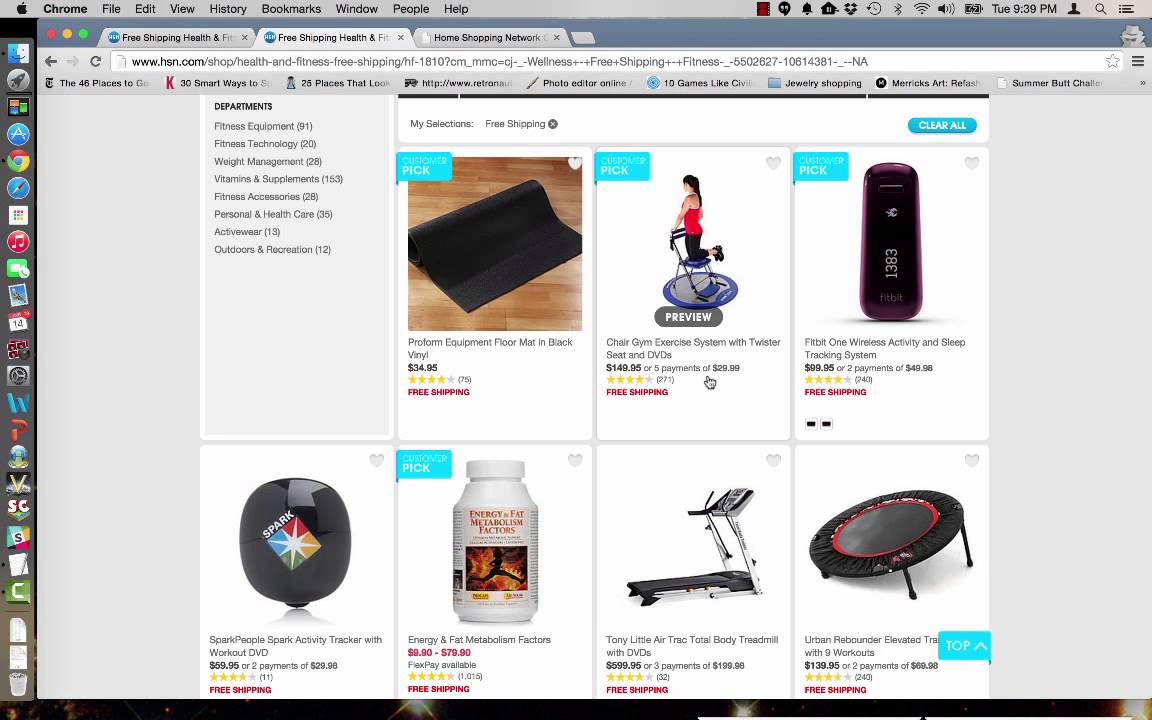A screenshot of a computer screen displaying a web browser window is shown. At the top of the screen, the browser's menu options are visible, including "Chrome," "File," "Edit," "View," "History," "Bookmarks," "Window," "People," and "Help." The bottom right corner of the screen shows the time as 9:30 p.m. on a Tuesday (TUE). 

The webpage currently open on the browser belongs to an online store, featuring various departments and a list of items for sale. The first item listed is a yoga mat priced at $34.95. The second item appears to be an ab workout device resembling a chair. The image depicts a woman on top of this device, with her knees bent and holding onto the top. This item is priced at $149.05, though the writing is quite small. Another item on the list is a technology device that resembles a Fitbit, priced at $90.95.